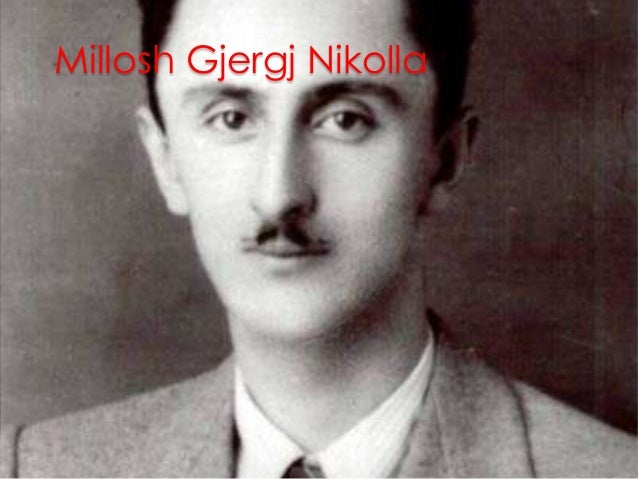This vintage black-and-white photograph, likely taken in the early 20th century, depicts a young, slender white man from his upper shoulders to his upper forehead, with the very top of his head and lower body out of frame. The man has dark hair and a notably prominent forehead. He is dressed in a dark business coat over a striped button-up shirt and a necktie. His eyes, framed by dark eyebrows, are looking intensely forward, matching the straightforward orientation of his body.

A thin, dark mustache rests on his upper lip, adding to the serious, neutral expression he holds. The background is solid gray, providing a stark contrast to the figure. Bold red text across the man’s forehead reads "Milosh Gjorg Nikola," though some variations in the name spelling occur in different captions provided. Despite the differing opinions on the exact era and name spelling, the photograph exudes a timeless, historical essence.